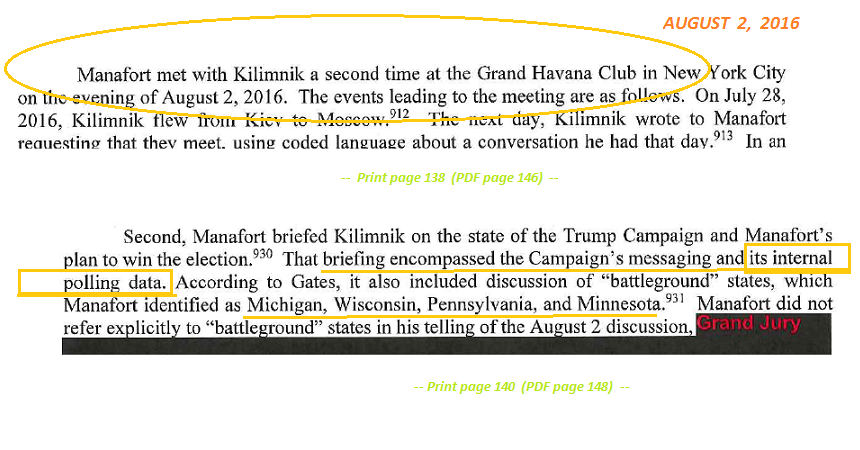The image is of a scanned document with a white background. In the top right corner, highlighted in orange text, is the date "August 2, 2016." The document appears to be an excerpt related to the Donald Trump campaign, specifically mentioning a second meeting between Manafort and Kilimnik at the Grand Havana Club in New York City on the evening of that date. The text highlights the events leading to this meeting, starting with Kilimnik flying from Kiev to Moscow on July 28, 2016, and subsequently writing to Manafort the following day, using coded language to request the meeting. The document details included in this excerpt are underlined and circled in yellow, with sections marked for emphasis. It mentions that Manafort briefed Kilimnik on the state of the Trump campaign, sharing internal polling data and discussing battleground states including Michigan, Wisconsin, Pennsylvania, and Minnesota. Additional notes in the document are written in green text, specifying "print page 138, PDF page 146," and "print page 140, PDF page 148." In the bottom right corner, written in red text, is the designation "Grand Jury."